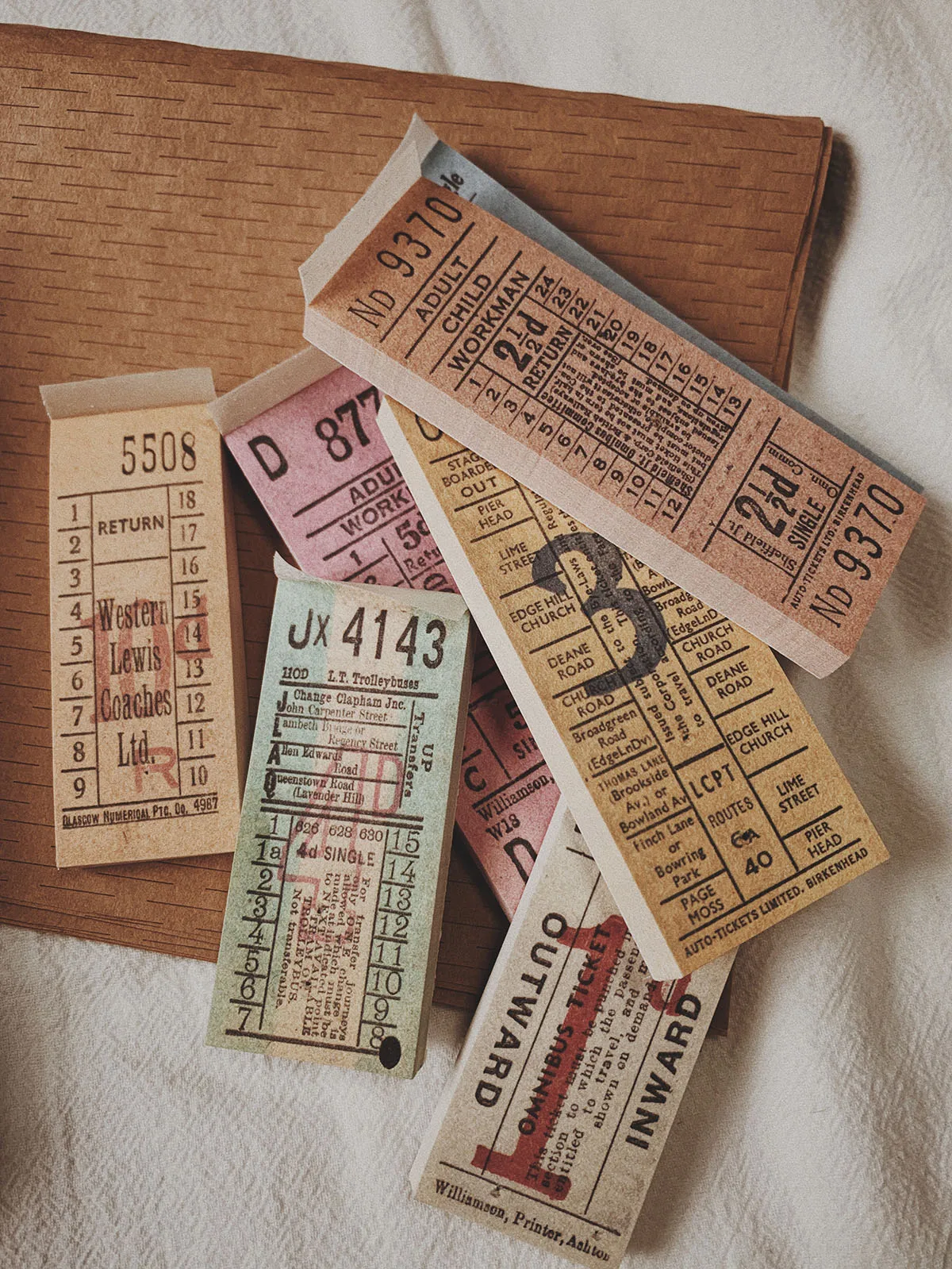In this vibrant overhead portrait photograph, the scene is set with a soft, fluffy white background, reminiscent of a bed sheet or towel. Resting on this white cloth is a prominently featured brown envelope, potentially made of cardboard or leather, and distinguished with darker brown dashes giving it a textured appearance. Scattered on top of the envelope are six variously colored ticket stubs, each about one inch wide and two to two and a half inches tall. The tickets display a range of muted hues including orange, red, yellow, blue, and green, and are organized in a somewhat haphazard pile. Each ticket sports unique numbers such as 5508, 5509, and so on, suggesting they could be parking tickets. Some tickets have more detailed inscriptions, like "NDN 9370," "adult," "child," "workman," and different usage charts, adding a layer of intricate detail to the arrangement.